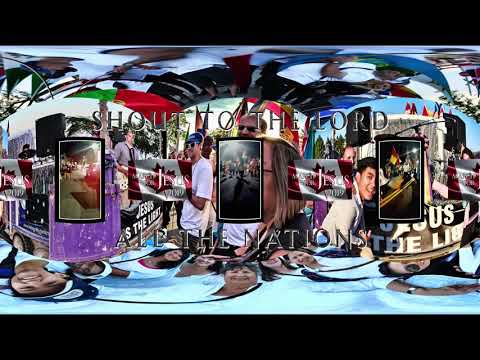The image is a collage of numerous photos, predominantly featuring people with a Christian theme. Text overlays prominently display the phrases "Shout to the Lord" at the top and "All the Nations" at the bottom. Additional text, "Jesus is the Light," appears against a black background, though some of the text is slightly warped and hard to read. 

The collage presents various religious photos and faces, with a noticeable central image of a person wearing a blue cap and sunglasses. Individuals in the collage are dressed in white t-shirts and jackets, some with dark hair. There is a noticeable event setting, possibly a table around which people are gathered, and some even appear to be holding a Canadian flag. 

The photo is marked by visual distortions, including black bars across the top and bottom, giving it a slightly warped, fragmented look. Despite these distortions, elements like the ceiling lights and the overall Christian imagery remain discernible amid the chaotic arrangement of faces and text.